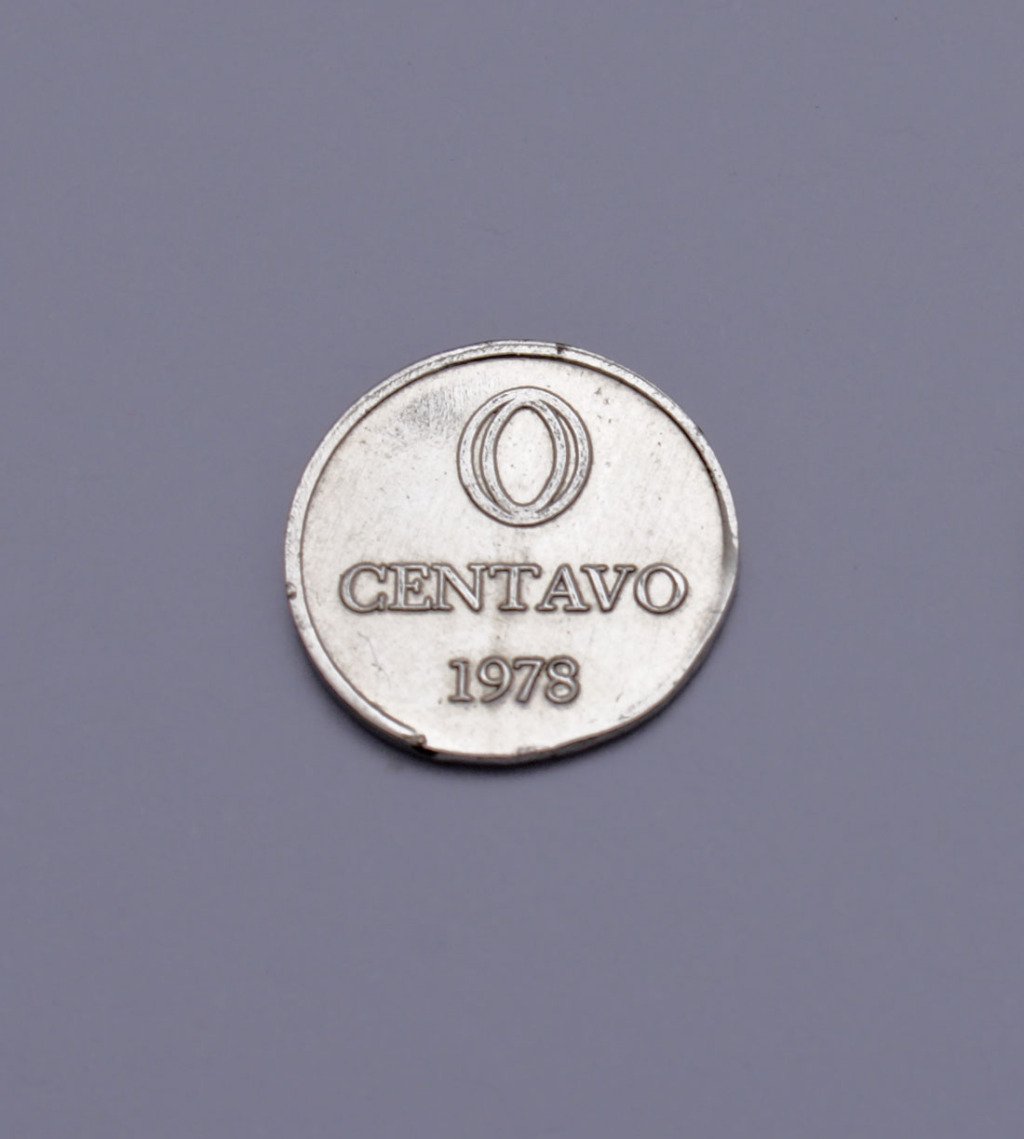The image showcases a well-worn old silver coin placed on a flat, dark gray surface, dominating the center of the photograph. The round coin features a raised edge along its border with prominent raised text in the center. At the top of the coin, there is a distinct '0' encased within a larger 'O'. Directly beneath, the word "Centavo" is inscribed in raised lettering, spelled out as C-E-N-T-A-V-O. Below this text, the date "1978" is clearly engraved. The coin's surface is marred with various scuff marks, dings, and chipped areas, indicating significant wear and tear, suggesting it has been extensively used or weathered over time.